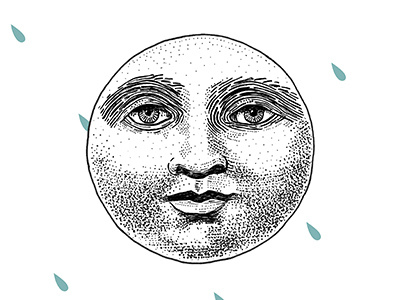This illustration features a stylized, anthropomorphized moon as the central focal point. The moon, depicted with pointillism and slight line work reminiscent of a woodcut design, displays intricate details such as deep eye sockets, a wide nose, and a subtle, closed-mouth smile. The facial features include very round eyes, puffy cheeks, and a pronounced chin, all crafted from an arrangement of dots and lines in black ink. The background is an opaque white, punctuated by six teal blue water droplets angled diagonally from the top left to the bottom right. One of these drops is partially cut off at the bottom edge, adding to the whimsical, vintage charm of the overall composition.